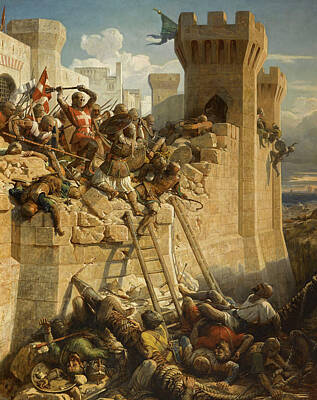The artwork is a highly detailed depiction of a medieval castle siege, potentially from the Crusades period, evident by the prominent knight in a red and white outfit bearing a cross. The scene is vividly colored with reds, whites, yellows, sandy grays, tans, and beiges. At the center of the chaos, a section of the castle wall has been breached, with a ladder propped against it. The focus shifts between the visceral conflict happening at the top of the wall, where armored men fiercely fend off the attackers, and the grim aftermath below, littered with the fallen. The painting captures various styles of armor, indicating a diverse group of warriors. In the background, additional towers of the sprawling castle suggest the extensive fortifications under siege. The composition of bodies, both in combat and lifeless, along with the turbulent action, conveys the intense and brutal nature of the medieval battle.